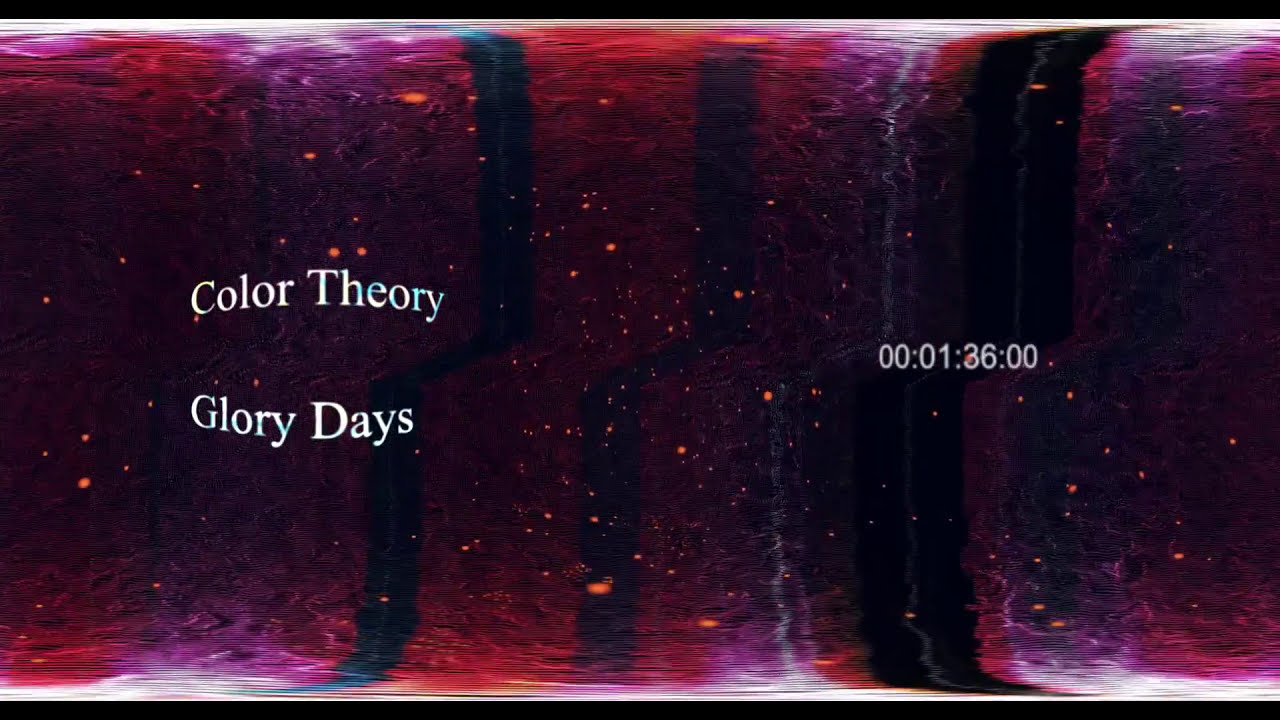The image is a wide horizontal rectangle presenting a blend of dark, rich colors, including deep burgundy, maroonish red, dark purple, and black, overlaid with white text. Thin black and white horizontal stripes frame the top and bottom edges of the image. The background has a jello-like consistency with vertical black streaks and scattered pink flecks, creating a liquid-like appearance. On the left side, in stretched, arching Times New Roman font, the white text reads "Color Theory Glory Days," with each word capitalized. On the right side, similar white text displays the numbers "00:01:36:00," suggesting a time code.